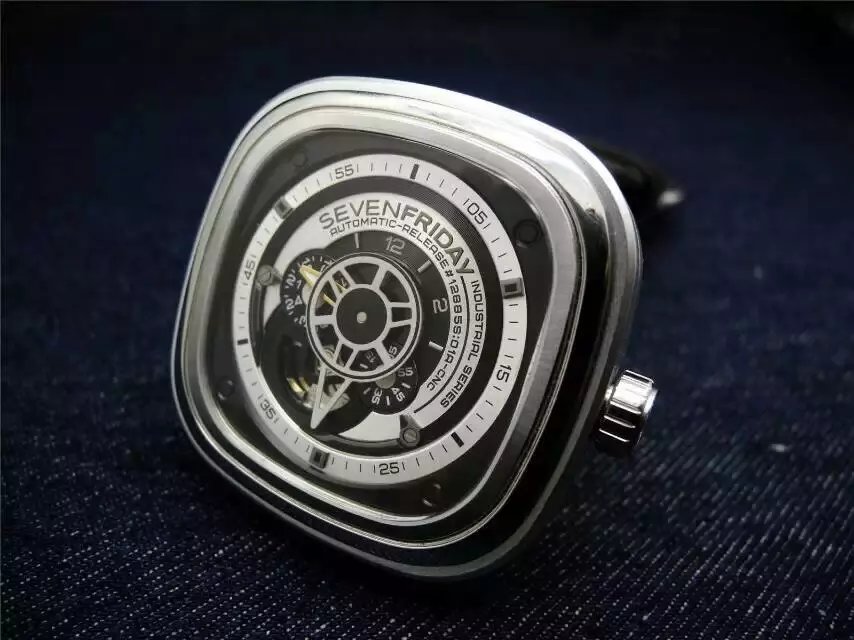This is a detailed and zoomed-in photograph of a sophisticated watch face. The watch has a distinctive design with the brand name "7 Friday Industrial Series Automatic" prominently sketched into its black and silver surface. The watch face features a unique layout, with the traditional 12-hour markings only partially visible – notably the 12, 2, and 5 – alongside detailed minute increments at 5-minute intervals (5, 15, 25, 35, 45, and 55). The watch is encased in silver metal with several interlocking circles, revealing the intricate gears and mechanisms inside, which give it a visually complex and industrial aesthetic. The watch face itself is encircled by a silver rim and includes a small dial on the side for adjusting the time. The background of the image is grey, enhancing the watch's dramatic appearance, and hinting at a slightly blurred black watch band.